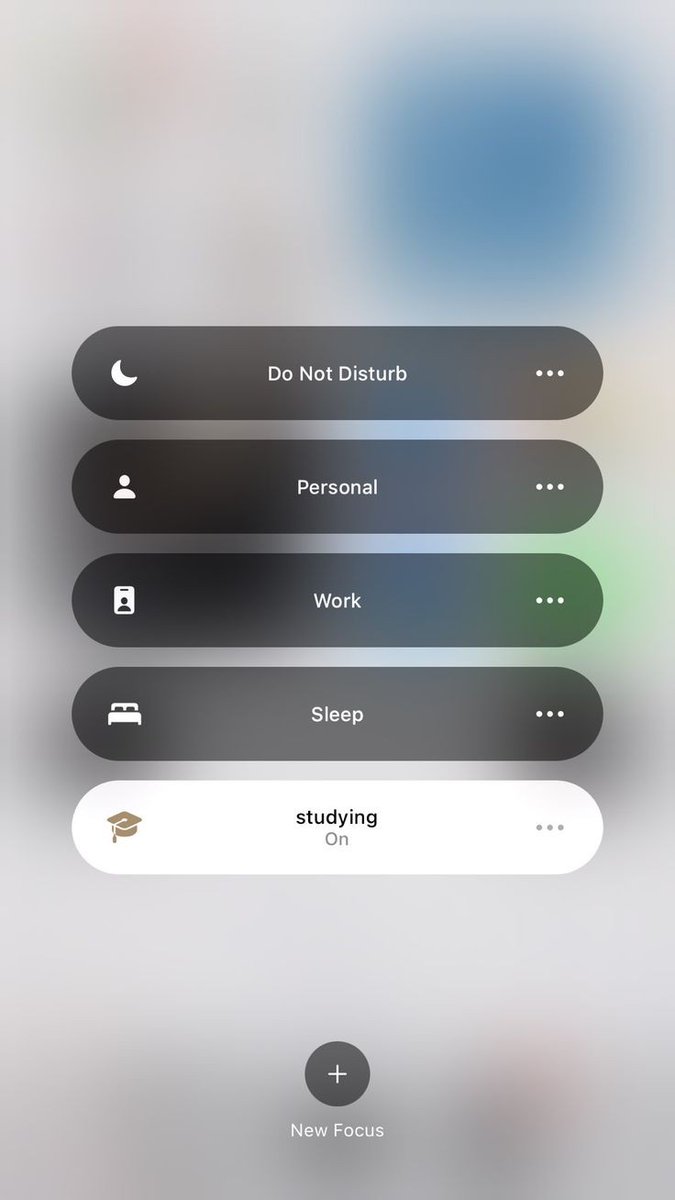The image features a screen capture from a mobile device with a silver background. In this background, faint blue circular shapes are noticeable towards the upper right corner, while dull gray blotches are scattered at the bottom. Displayed prominently on the screen are five notifications, each contained within an elongated horizontal oval frame. The top four notifications have a gray background, while the fifth has a white background. The notifications are listed as follows from top to bottom: "Do not disturb," "Personnel," "Work," "Sleep," and "Studying on."